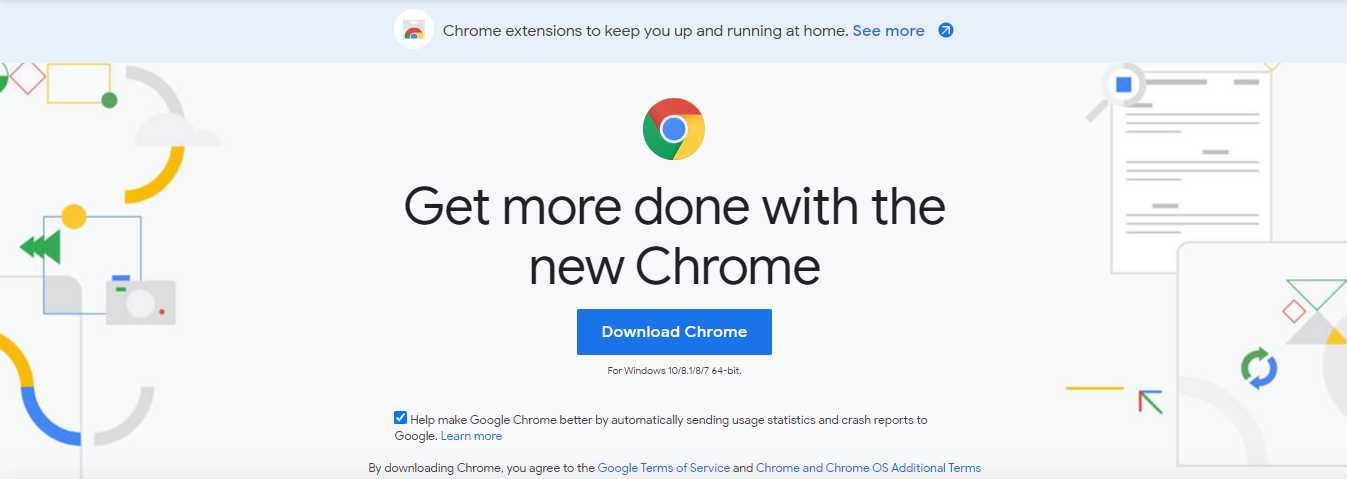In this image, we see a Google Chrome promotional screen. The top of the screen features a light gray background with the text, "Chrome extensions to help keep you running at home," followed by a "See More" link. Directly below this is the iconic Google Chrome logo. Underneath the logo, a bold black text proclaims, "Get more done with the new Chrome." A prominent blue rectangle below this text displays a call-to-action button labeled "Download Chrome."

Proceeding further down, there is some very small, hard-to-read text, likely containing additional information or disclaimers. This is followed by more diminutive text in a mix of blue and black colors.

The left side of the screen showcases a decorative design featuring several curved lines and shapes: three gray lines, a single blue line, two yellow lines, a sideways green tree shape, and a yellow circle.

On the right side, there's an illustration of a piece of paper with three sentences written on it. In the bottom right corner of this illustration, there's a square-like shape. Adjacent to it are a green arrow and a blue arrow pointing towards an hourglass-shaped icon. The bottom half of this hourglass icon is gray, while the top half is white. An additional arrow is positioned to the left of this design in the bottom right corner.

The rest of the image is set against a clean, white background, creating a minimalist and modern appearance. This thoughtful layout effectively highlights the features and benefits of Google Chrome, encouraging users to download and utilize the new browser version.